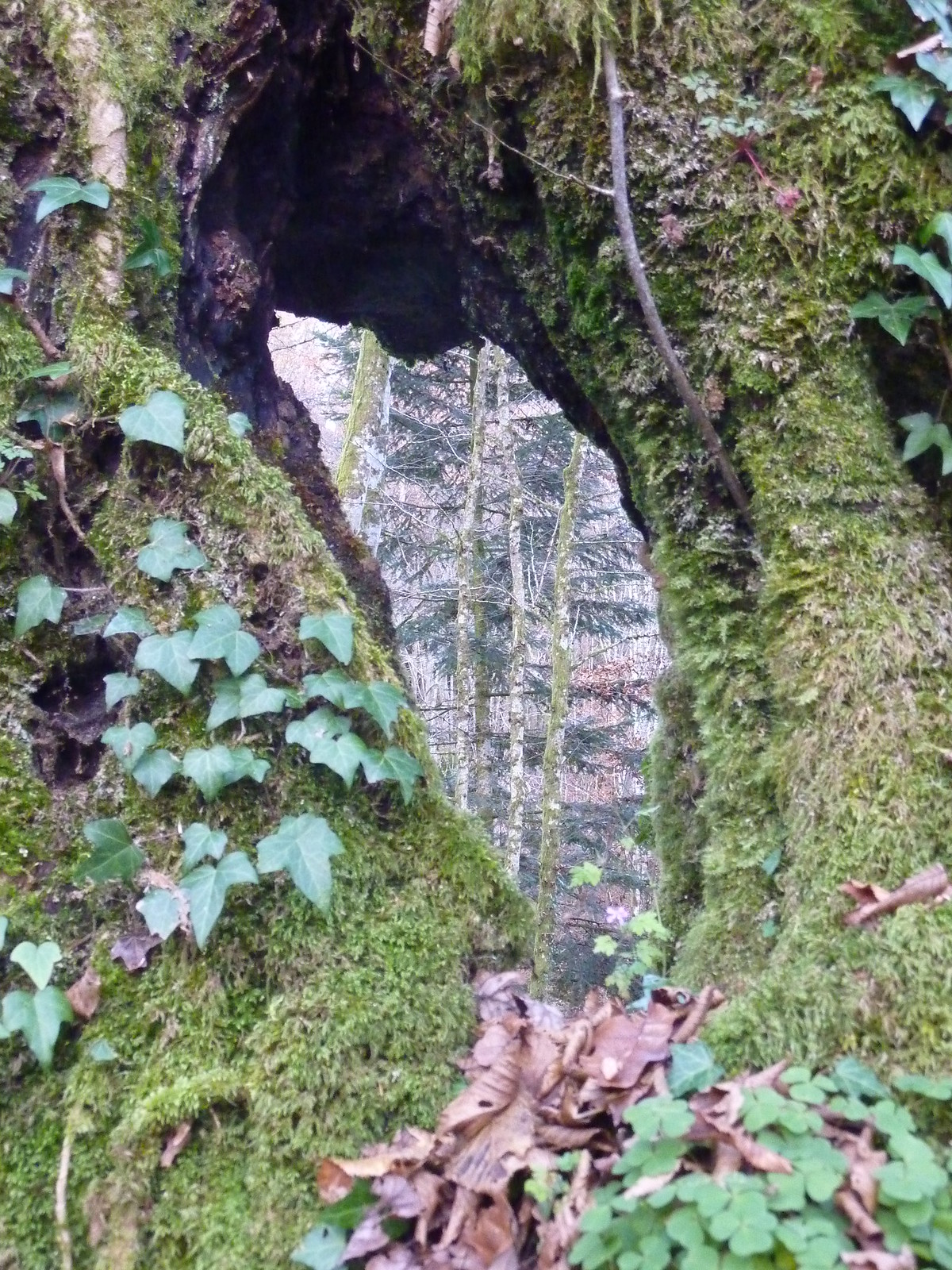The image presents a mesmerizing outdoor nature scene featuring a towering, moss-covered arch formed by two intertwined tree trunks. This natural structure, approximately 30 feet high, is draped in lush green moss, ivy, and vines, creating an almost whimsical, tunnel-like passage. The archway's opening, centrally positioned and slightly veering right at the bottom, reveals a darker interior that contrasts sharply against the backdrop. Beyond the arch, a sunlit forest with towering trees, possibly including a fir, stretches into the distance, adding depth to the scene. The ground in the foreground is a mix of green and dried brown leaves, alongside various plants and weeds nestled in the nook where the trunks meet. The scene is brimming with greenery and woodland elements, embodying the essence of a serene, wooded forest.